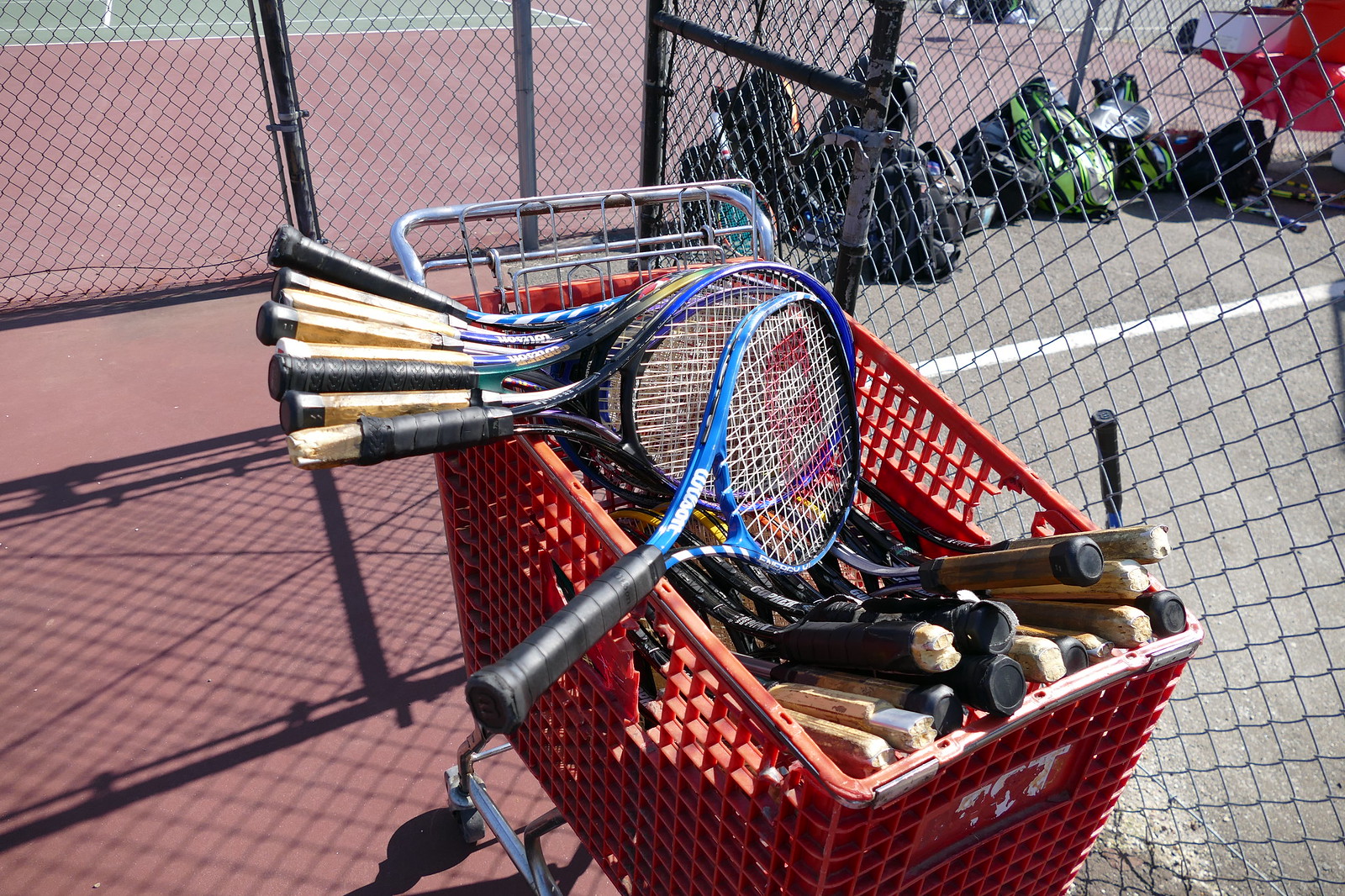The image depicts a detailed scene on a tennis court with a distinct division of colored surfaces— a reddish clay-like surface on the left side and a green surface on the right, continuing into the background. Surrounding the courts is a fence that runs along the bottom-left corner and separates different sections. Dominating the center of the photograph is a red plastic shopping cart with a metal handle and wheels. The cart is filled with dozens of tennis rackets, some of which are jutting outward, especially toward the right. In the background, leaning against one of the fences, there are numerous bags and backpacks, typical of what players might bring to the court for storing their rackets and tennis balls.